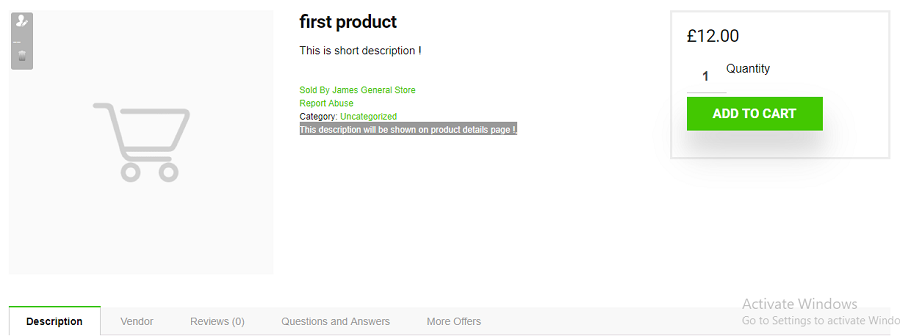This is a detailed view of a shopping website interface displayed on a computer screen. On the left side of the screen, there is a large square with a gray background. At the top of the interface, a gray banner contains account-related information, including an icon of a shopping cart.
To the right, the main display area features a white background. The central section is dominated by the title "First Product," and below it, a brief description stating, "This is a short description." Further down, in green text, the product is noted as being sold by "James, General Store" with options to "Report Abuse" and a category marked as "Uncategorized."

A gray banner underneath mentions, "This description will be shown on the product details page." Adjacent to this banner, a box displays the price as "£12," indicating British pounds, and a quantity selector set to one unit. Beside it, a green "Add to Cart" button is prominently placed.

At the bottom of the screen, there are several tabs, including "Description," "Vendor," "Reviews" (with a zero review count indicated), "Questions and Answers," and "More Offers." The "Description" tab is selected, highlighted with a green line above it. On the bottom right corner of the image, there is a message prompting to "Activate Windows," instructing the user to go to settings to complete activation. The bottom section of the screen shares a gray coloring similar to the shopping cart area, maintaining a consistent design aesthetic.